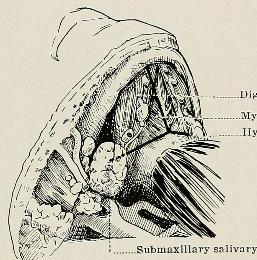This image is a detailed black and white sketch that appears to be from a scholarly textbook, featuring a close-up diagram of a body part. The diagram is printed on a white background and prominently includes labels and arrows, highlighting specific areas of interest. At the bottom of the sketch, the term "submaxillary salivary" is clearly indicated, suggesting the illustration is focused on anatomical structures related to the mouth. Toward the top right, several partially visible labels are cut off, reading "DIG," "MY," and "ILY." The diagram appears to include cross-sectional views, showing intricate inner structures that resemble both muscular and glandular elements, depicting what seems to be an anatomical part rather than a plant or fruit. The detailed depiction of the internal composition hints at a section of the mouth, possibly the salivary glands.